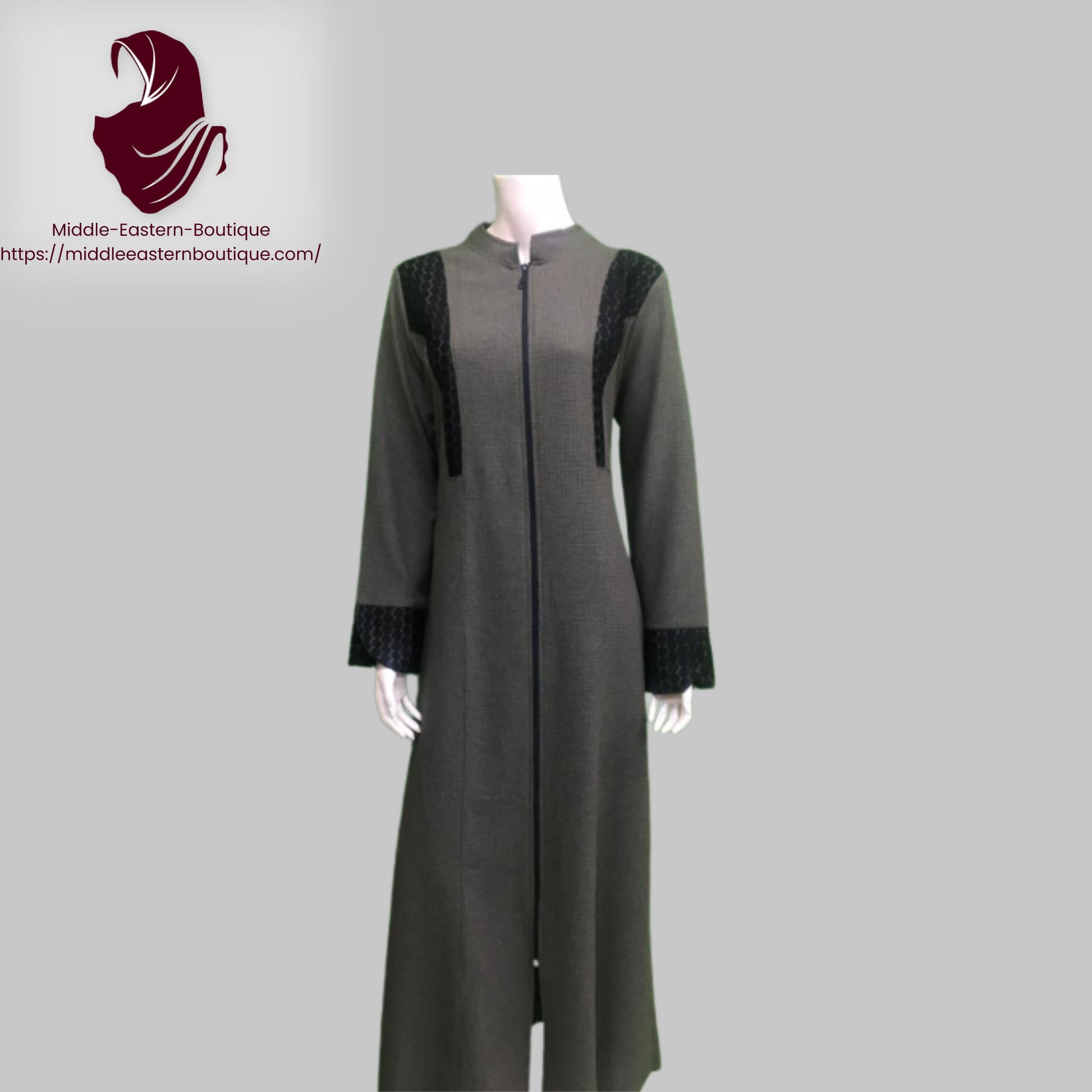The image displays a headless mannequin dressed in a long, ankle-length, dark gray garment resembling a kimono. The dress, likely made of thick cotton or wool, features a centrally placed zipper running from top to bottom. The sleeves are long, each ending in black cuffs adorned with a subtle paisley design. This paisley pattern repeats on two black appliques that stretch from the shoulder down to the chest area, adding a touch of elegant symmetry. The dress sports a modest high collar, distinctly avoiding the turtleneck style. The background is a light gray, and in the top left corner of the image, a logo depicting a red turban or scarf is visible, accompanied by the text "Middle Eastern Boutique" and the URL "https://middleeasternboutique.com". This setup suggests a sophisticated, traditional Middle Eastern overcoat with intricate detailing.